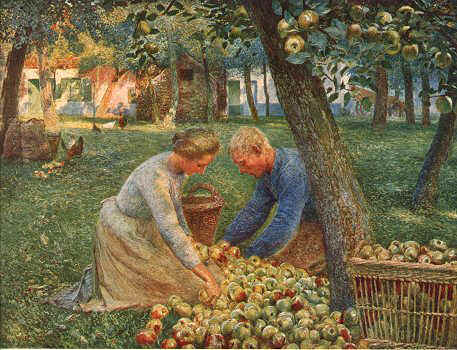This detailed oil painting captures a serene scene of a man and a woman gathering apples in an abundant orchard. Both subjects are kneeling on lush green grass, beneath a tall apple tree whose branches are heavy with green and red apples. The woman, whose grayish hair is tied back, is wearing a long-sleeved gray dress paired with a yellow apron. She leans over to collect apples and places them into a brown wicker basket behind her. Across from her is the man, dressed in a blue long-sleeved shirt and brown pants, similarly engaged in gathering apples. His hair is similarly grayish. Surrounding them, scattered on the ground, are numerous apples, some of which have already been piled into a basket in the lower right-hand corner. The background reveals more apple trees and a couple of houses, adding depth to the orchard setting. The overall color palette is dominated by various shades of green from the trees and grass, emphasizing the lushness of the scene. The painting’s impressionistic brushstrokes add a slightly blurry yet charmingly detailed texture to the image, enhancing the tranquility of this pastoral moment.